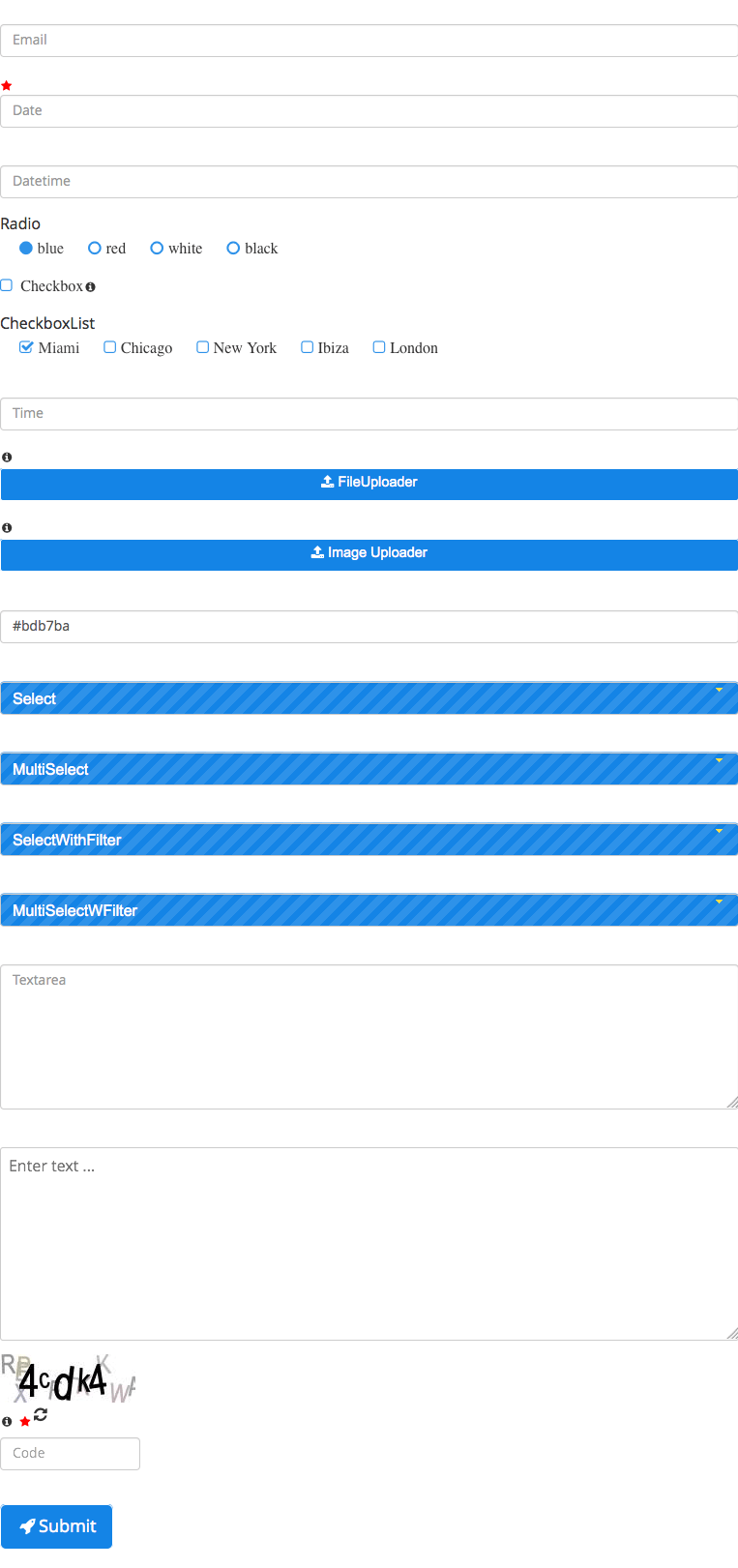The image depicts a detailed form layout, likely designed for data collection, possibly for a mobile application due to its horizontal orientation. 

At the top of the form, there is a field labeled "Email" where users are prompted to type their email address. Following this, there are fields for "Date" and "Daytime." Below these fields, there is a radio button section with options: blue (selected), red, white, and black.

Next is a series of checkboxes. The category starts with "Miami," which is checked, followed by options for Chicago, New York, Ibiza, and London. Under these, there is a "Time" field, followed by a "File Uploader" and an "Image Uploader."

Further down, a section that is not clearly legible is present, followed by a "Select" dropdown menu, a "Multi-Select" dropdown menu, a "Select with Filter" option, and a "Multi-Select with Filter" option. There is also a Textarea box labeled "Textara" and another box prompting users to "Enter Text." Additionally, there is a CAPTCHA box to verify that the user is human.

At the very bottom of the form, there is a prominent blue "Submit" button. The overall layout suggests that the page is designed to gather a variety of user inputs, including personal details and file uploads.